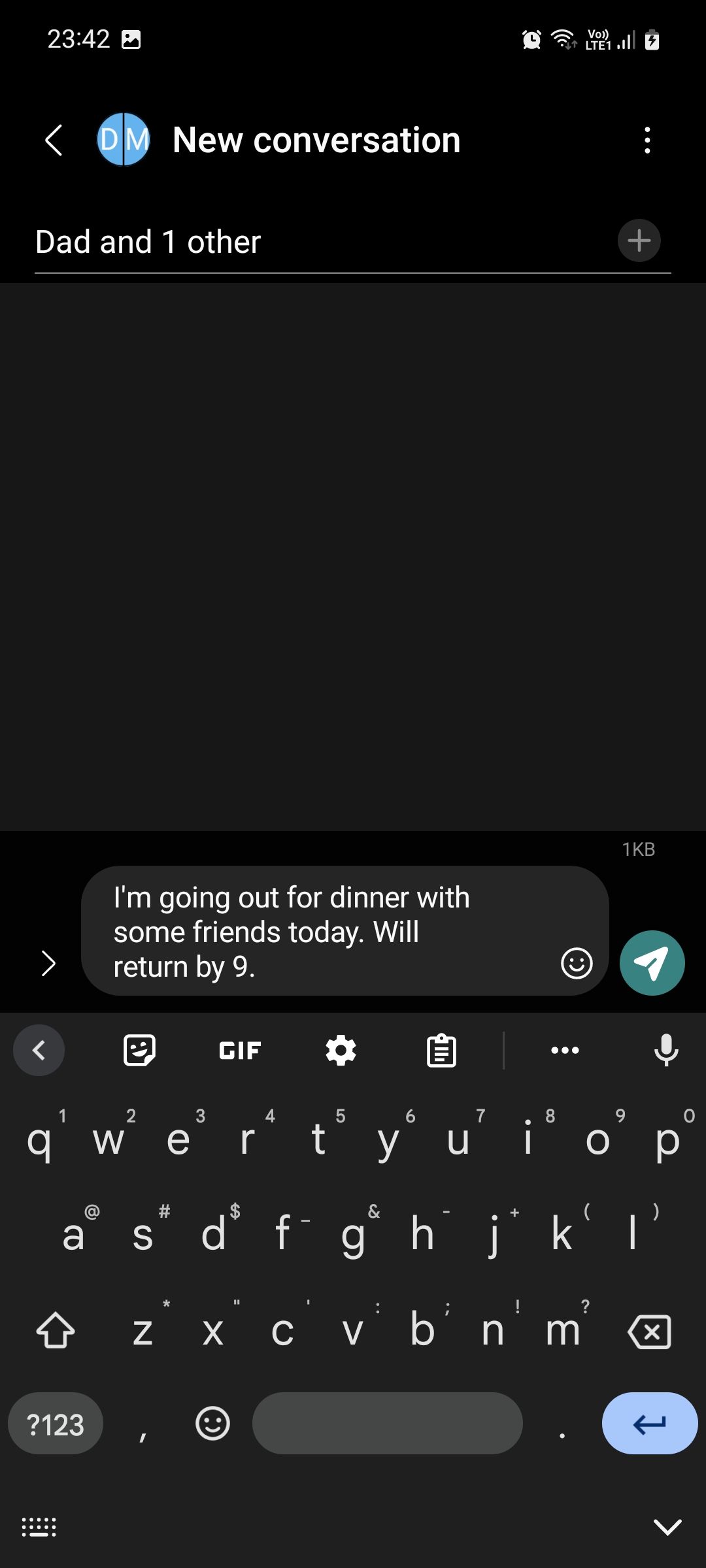The image depicts a phone screen taken at 11:42 PM, as shown by the clock on the top. The phone has LTE connectivity with good signal strength and a fully charged battery. The screen displays a chat interface with a black background. At the top, there is a blue circle bisected by a black line, with the letter "D" on one side and "M" on the other. The chat window is titled "New Conversation" with "Dad and One Other" participants.

The message in the text box reads: "I'm going out for dinner with some friends today, we'll return by nine o'clock." Following the text is a happy face emoji. Below the text box is a green button for sending the message. The keyboard is visible at the bottom of the screen, featuring a microphone icon on top, alongside a clipboard and settings button. Additionally, there is a back arrow and a "1, 2, 3" button with a question mark for switching between keypad modes.